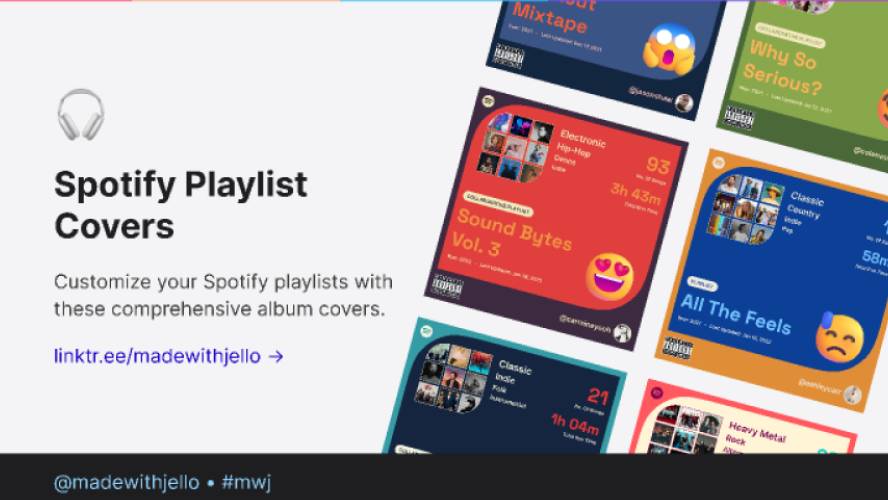This image captures a screenshot from a website interface designed to customize Spotify playlists. On the left side, a grey background features black text announcing "Spotify playlist covers" accompanied by a grey headphone infographic. The text encourages users to "Customize your Spotify playlist with these comprehensive album covers." Below this section, a blue hyperlink reads "linktr.ie/madewithjello," followed by a forward arrow symbol. 

Immediately beneath this, a black band displays grey text that says "madewithjello #nwj." 

The main content on the right showcases six distinctive album cover designs arranged in two rows of three. Starting from the top left, the first cover is blue with the title "Mixed Tape," featuring an alarmed-looking emoji. Next, the green cover with "Why So Serious?" shows the partial edge of an unseen emoji. The red cover, "Soundbites Volume 3," features an array of smaller album cover thumbnails with a smiling emoji with heart eyes at the center. 

On the second row, the first cover is a combination of blue and yellow, titled "All The Feels," adorned with a sad crying emoji. Similar to the previous row, this cover is overlaid with a grid of smaller song covers. The dark blue cover simply titled "Classic" also incorporates this grid pattern. Lastly, the red and cream cover titled "Heavy Metal" bears a grid of nine smaller images, although only six are discernible and too small to identify clearly.